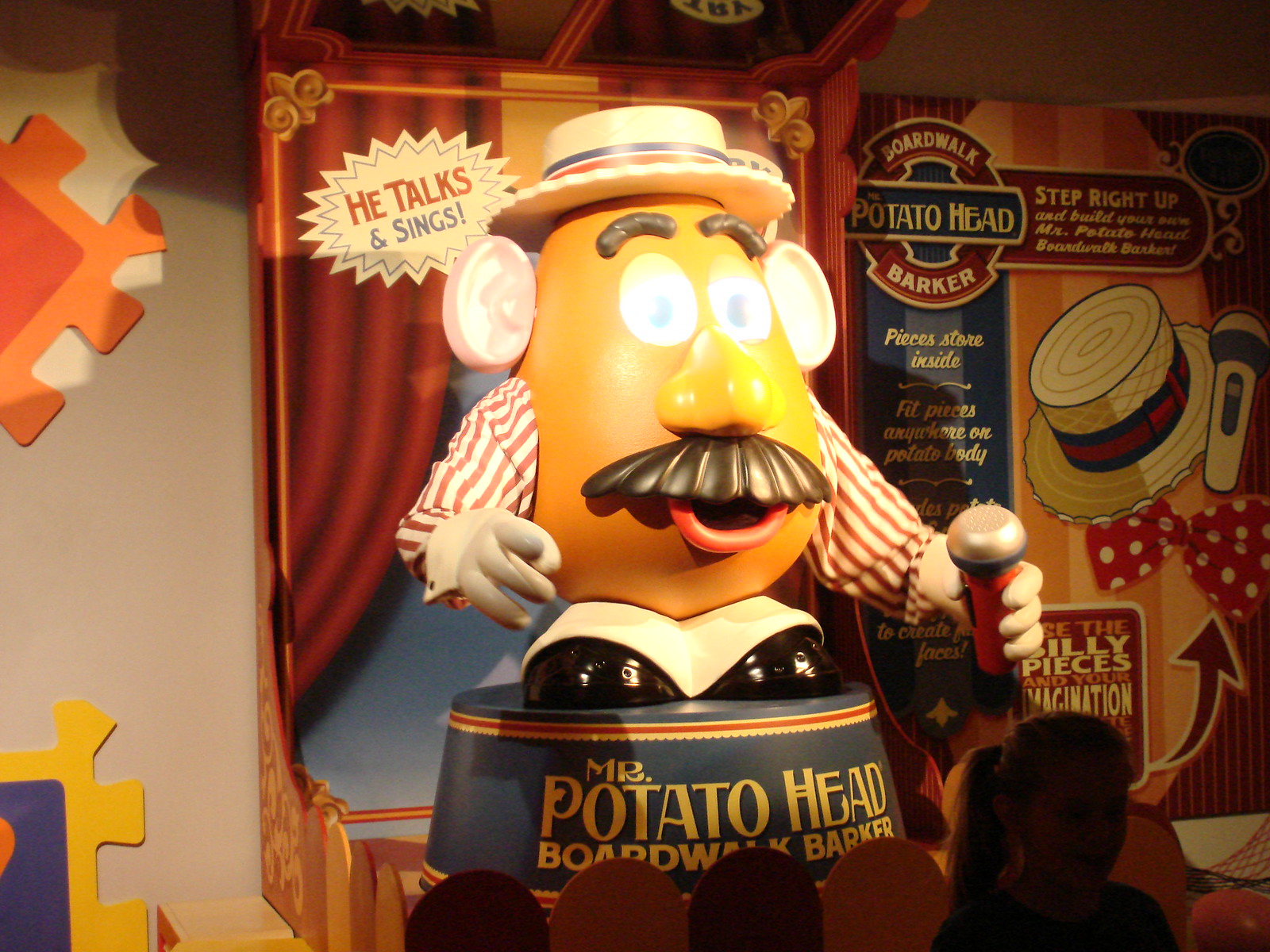The image depicts a large Mr. Potato Head statue, standing approximately three to four feet tall, inside what appears to be a museum or an interactive display. The dark room is illuminated by Mr. Potato Head, highlighting its detailed features. He wears a straw-brimmed hat adorned with red, white, and blue bands, matching his vertically red and white striped sleeves. Mr. Potato Head holds a microphone in his right hand and stands atop a podium labeled "Mr. Potato Head Boardwalk Barker" in yellow text on a blue background. Behind him, colorful banners and signs, including one that reads "Step Right Up" and another stating "He talks, he sings," reinforce the interactive aspect of the display. A figure of a young girl with a ponytail is partially visible in the bottom right, providing a sense of scale. The setting is completed with a backdrop of puzzle pieces and balloons, suggesting a playful, child-friendly environment.